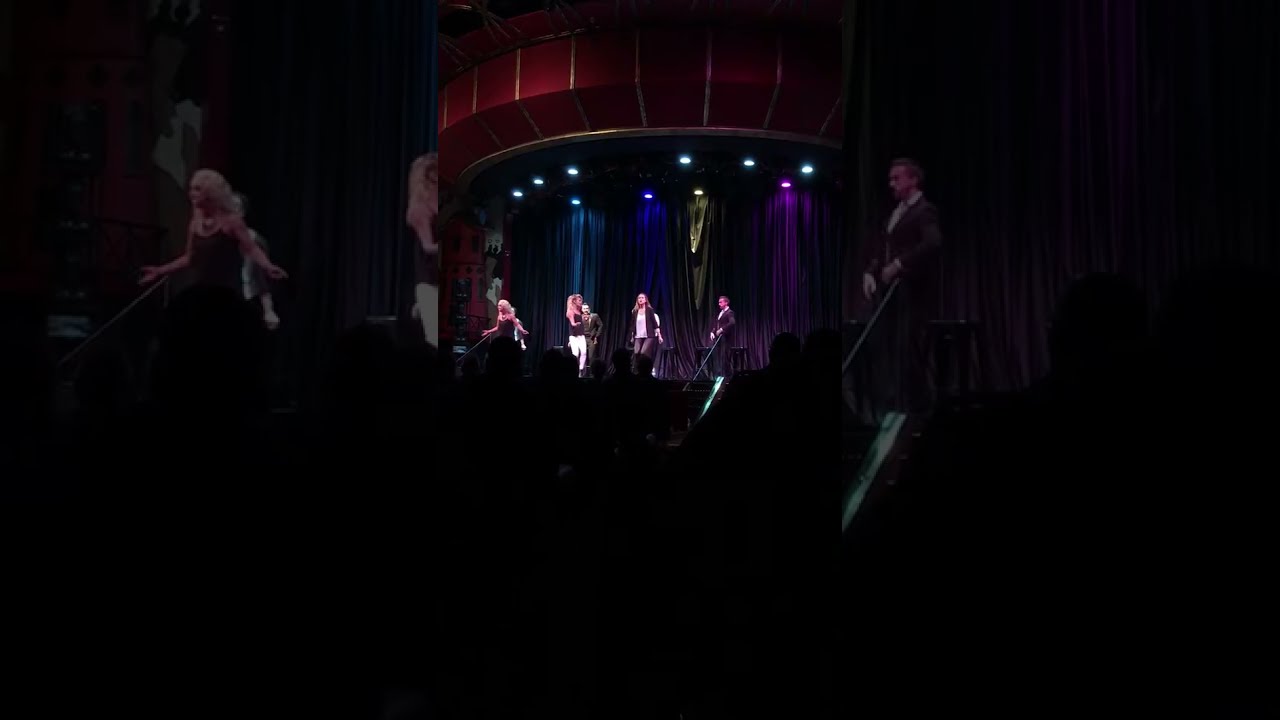The photograph captures a live performance on a brightly lit stage featuring a group of six individuals. The background is adorned with cascading curtains tinted in shades of teal, blue, and gold, illuminated by vibrant spotlights from above, casting hues of blue, light blue, yellow, and purple onto the scene. At the center of the stage, multiple women are dressed in black attire paired with jeans or pants, except for a few in white and black outfits. A woman in the middle stands out in a black jacket and white blouse, possibly singing or dancing, while another woman, similarly outfitted, is positioned on the side. There are also a couple of men on stage; one in a black suit is notably in motion. Some performers utilize head-mounted microphones, hinting at a vocal performance. The stage features a set of stairs with a railing, adding depth to the setup. At the forefront of the image, the audience appears as black silhouettes, their presence implied rather than detailed. The edges of the image are framed by black bars, focusing attention on the dynamic scene within.